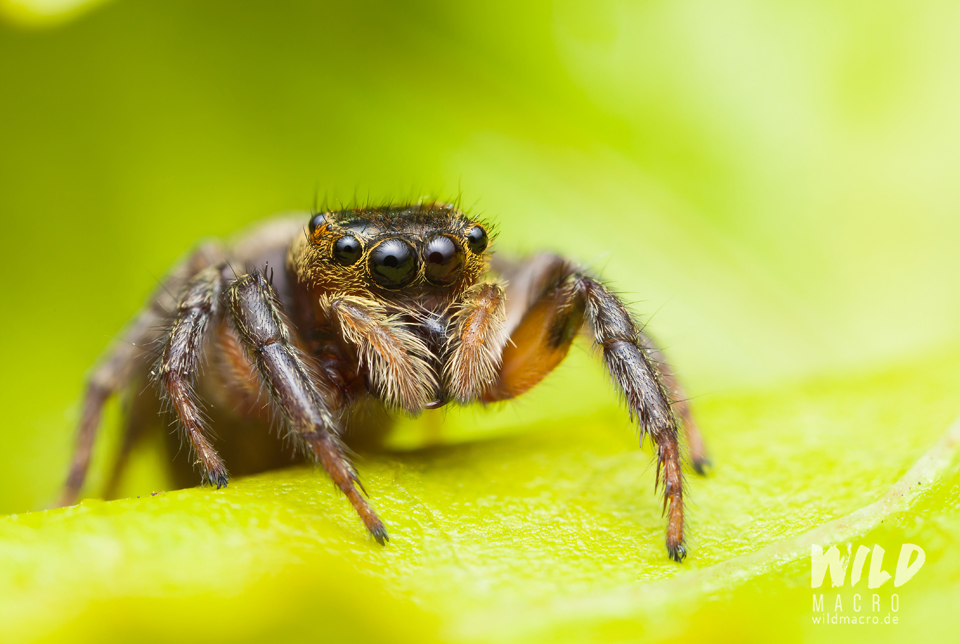This close-up photograph captures a meticulously detailed image of a brown, hairy spider situated on a vibrant, lime green leaf. The spider's face is clearly in focus, revealing a fascinating arrangement of six jet-black eyes that resemble black pearls, with two large ones centrally positioned and smaller ones spaced out on either side of its head. The spider’s mandibles, located at the front, are also covered in brown hairs. The spider has a black head with short hair, and its dark brown legs become progressively lighter towards the tips. The back legs are blurred, emphasizing the spider's frontal features. The surface of the leaf beneath the spider appears waxy and yellowish, enhancing the contrast with the spider’s dark coloration. In the bottom right corner of the image, a watermark reads “wild macro” with “wild macro dot D E” beneath it. The spider, placed slightly to the left of center, strikes an imposing figure despite its small size, creating a captivatingly detailed and somewhat eerie visual.